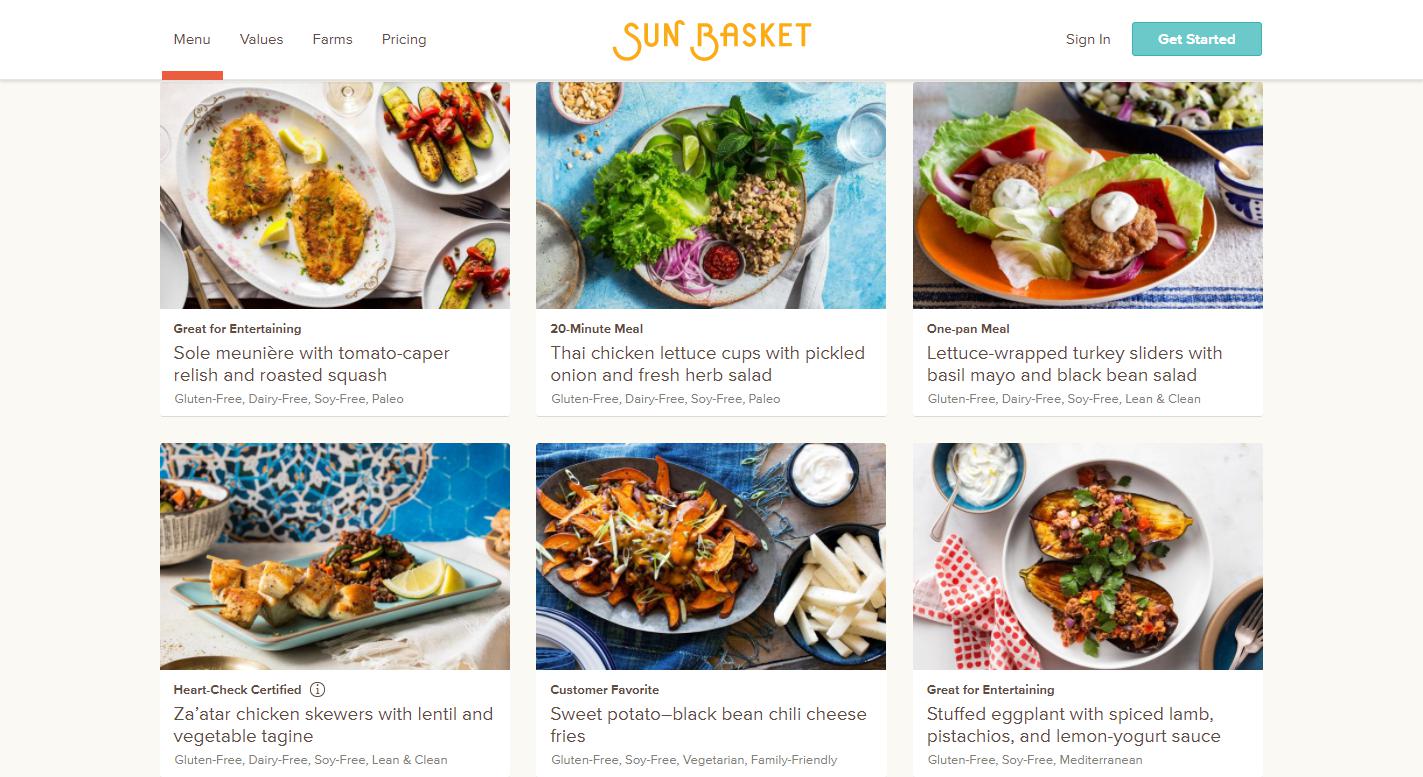This image is a detailed screenshot of an app or website for a food blog, possibly a recipe browser called "Sun Basket". The interface features a white navigation bar at the top. On the left side of this bar, there is a navigation menu with items such as "Values," "Farms," and "Pricing." Currently, the "Menu" item is selected, indicated by a thick red underline. 

Centrally located in the navigation bar is the "Sun Basket" logo, presented in a golden yellow color with a somewhat ornate font, particularly noticeable with the stylized "S" and "B." On the right side of the navigation bar is the user area featuring a "Sign In" link and a prominent, blue, rounded button labeled "Get Started."

Below the navigation bar, the main section is divided into a light gray background grid composed of three columns and two rows, forming six individual tiles. Each tile showcases a different recipe, with an image, a heading, an excerpt, and relevant tags.

For instance, the first tile displays a top-down view of a dish that appears to consist of breaded salmon or fish slices in an oval bowl with a floral pattern. Accompanying this are sliced vegetables with a red garnish on a separate plate. The title below the image reads "Great for Entertaining," with an excerpt in another language, "soul manure with tomato keeper relish and roasted squash." The tags for this recipe include "Gluten-Free," "Dairy-Free," "Soy-Free," and "Paleo," among others.

The succeeding tiles follow a similar format, each highlighting different food items, descriptive excerpts, and specific dietary tags.